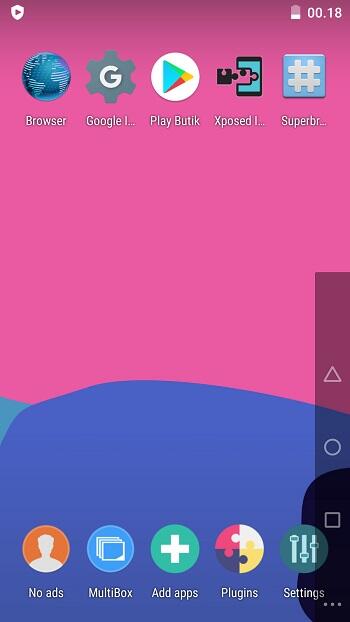Here is a cleaned-up and detailed caption for the image described:

---

Screenshot of an Android smartphone's app drawer. In the upper left corner, there is a shield icon with a play button on a pink background. The top right corner displays the battery level at approximately 25% and the time as 00:18, likely indicating 12:18 AM for those using a 12-hour clock. 

The app drawer features:
- A blue icon with a globe labeled "browser" in white.
- A blue gear with a white "G" labeled "Google L" in white text.
- A white icon with a blue, red, and yellow triangle labeled "Play Butik."
- An app with an icon of a phone with a puzzle piece missing, labeled "Exposed."
- A square icon with a hashtag labeled "Super BR."
- An orange icon with the silhouette of a person labeled "No Ads."
- A light blue icon with document-like graphics labeled "Multi Bots."
- A teal icon with a white plus symbol labeled "Add Apps."
- An icon with puzzle pieces in blue, black, yellow, and white labeled "Plugins."
- An icon with sliders on a gray background labeled "Settings."

At the bottom of the screen, there are app navigation controls including a triangle, a circle, and a square, alongside three vertical dots on a gray background in the bottom right corner.